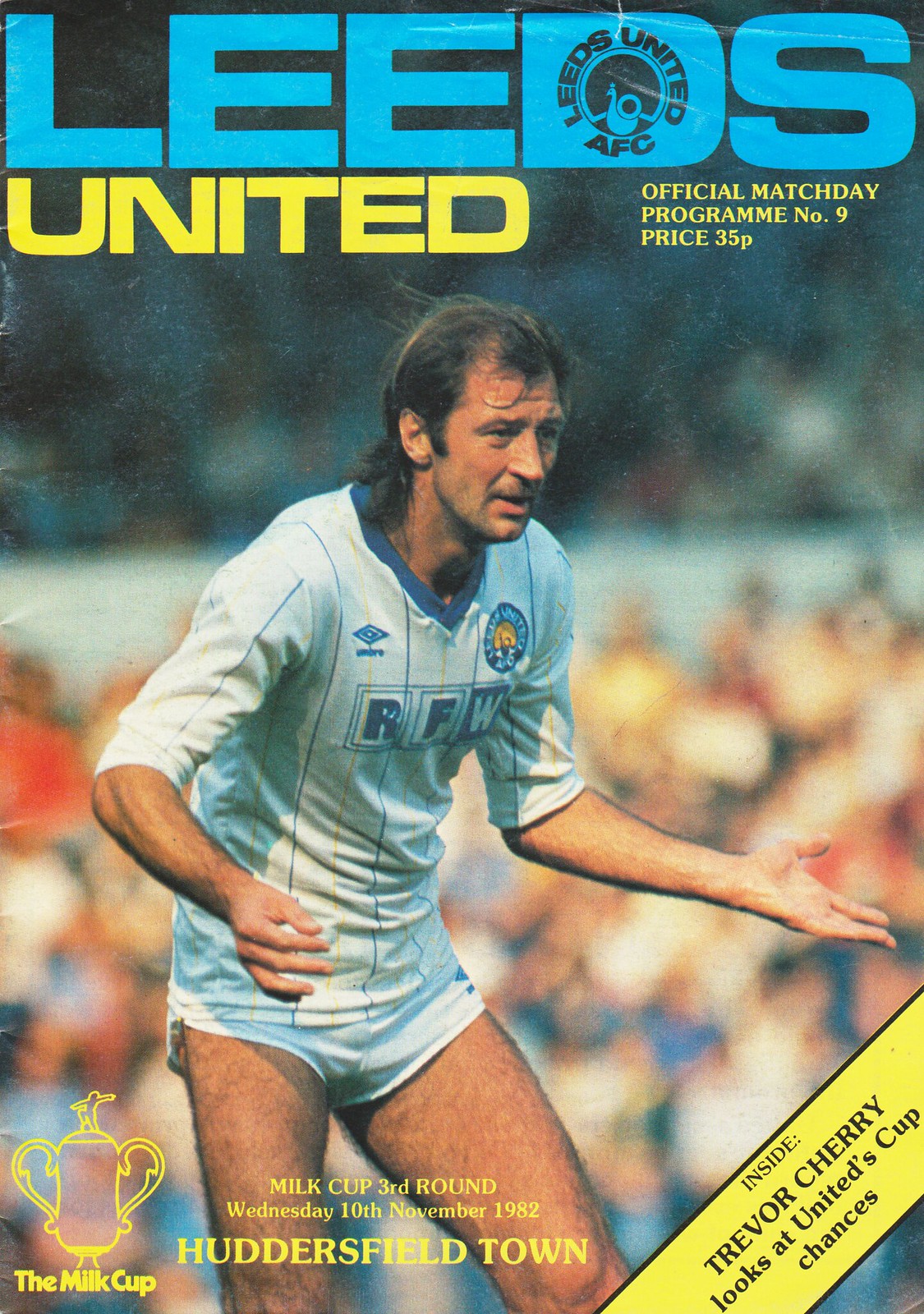The cover of the Leeds United official match day program from Wednesday, November 10, 1982, prominently features a male soccer player dressed in the team's uniform. He is wearing short white shorts and a white shirt adorned with vertical blue and yellow pinstripes that extend to his elbow-length sleeves. The player's hands are outstretched and his knees are bent as if he is ready to engage in the match, possibly in a goalkeeper's stance. On the left side of his chest is a blue and yellow circular team symbol, while the right side displays the Umbro logo. Surrounding him, the background displays the blurred image of a densely packed crowd, creating a vibrant atmosphere.

The top of the program reads "Leeds United AFC," with "Leeds" in bold blue letters and a stylistically colored 'D', and "United" beneath it in bright yellow text. Just beside "United" in a smaller font, it states "Official Match Day Program Number 9, Price 35p." The bottom left corner of the cover highlights the "Milk Cup Round 3" with an outline of a trophy next to the text along with the match date, "Wednesday, 10th of November, 1982," against Huddersfield Town. Adjacent to this, the program teaser "Trevor Cherry looks at United's Cup chances" is written in yellow text over a stripe.